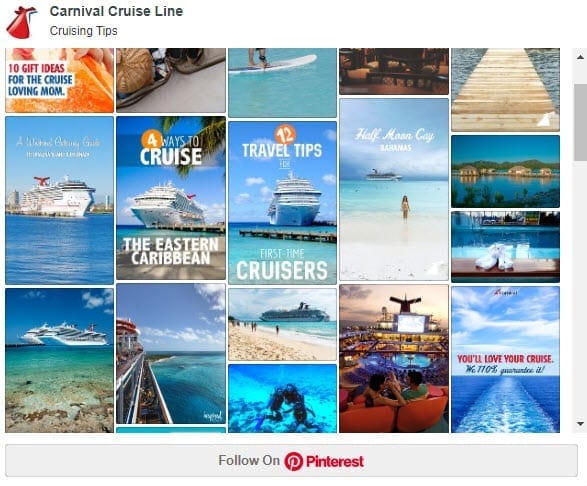This is a detailed screenshot of a Carnival Cruise Line promotional page. In the top-left corner, the recognizable Carnival Cruise Line logo is visible, resembling a red party hat with a bell-like design. Directly beneath the logo, the text "Cruising Tips" is displayed prominently. The main section of the image is filled with various smaller sections and article previews.

At the top left, there's a banner titled "10 Gift Ideas for the Cruise Loving Mom," followed by a repetitive layout of images featuring luxurious, giant white cruise ships. However, the text on these ships is largely illegible due to the low image quality. 

In the bottom left, another image from a different angle shows a cruise ship viewed from the shore, situated on a beach. Surrounding this image are additional article titles such as "Four Ways to Cruise the Eastern Caribbean," "12 Travel Tips for First-Time Cruisers," and "Half Moon Cay, Bahamas," suggesting a collection of informative articles tailored for both new and experienced cruisers. At the bottom right, there's a motivational caption that reads, "You'll Love Your Cruise," enhancing the page's welcoming and informative appeal.